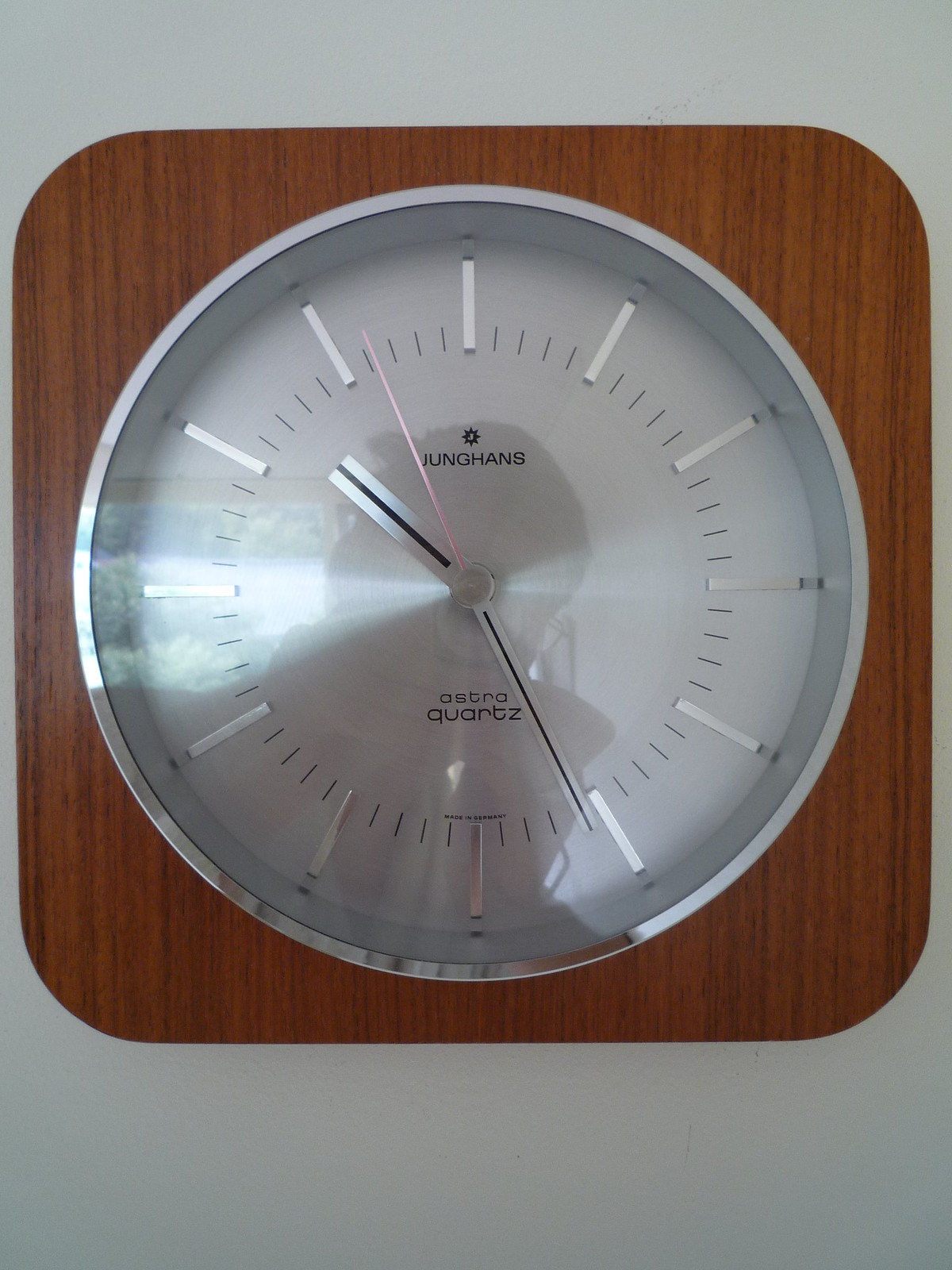This is a detailed close-up photograph of a modern, Scandinavian-style wall clock, elegantly mounted on a medium to dark brown wood grain square with slightly rounded edges, resembling a walnut cutting board. The clock itself is the centerpiece, featuring a sleek silver frame with a reflective glass face. The face is silver with minimalist design elements: no numerical numbers, only silver lines to denote the hours, with every fourth line slightly elongated. It has three hands—a short, flat silver hour hand, a longer, thin minute hand, and an even thinner red sweep second hand.

Prominently displayed on the top of the clock face is a small sun-like symbol and the word "Junghans" in black lettering, with the word "Astroquartz" positioned underneath. Reflecting off the clock's glass surface is the image of a young man capturing the photograph, likely using an iPhone. The clock contrasts with the white wall, which surrounds the photograph's upper, left, and right borders slightly and extends about two inches at the bottom, emphasizing the clock's modern aesthetic.